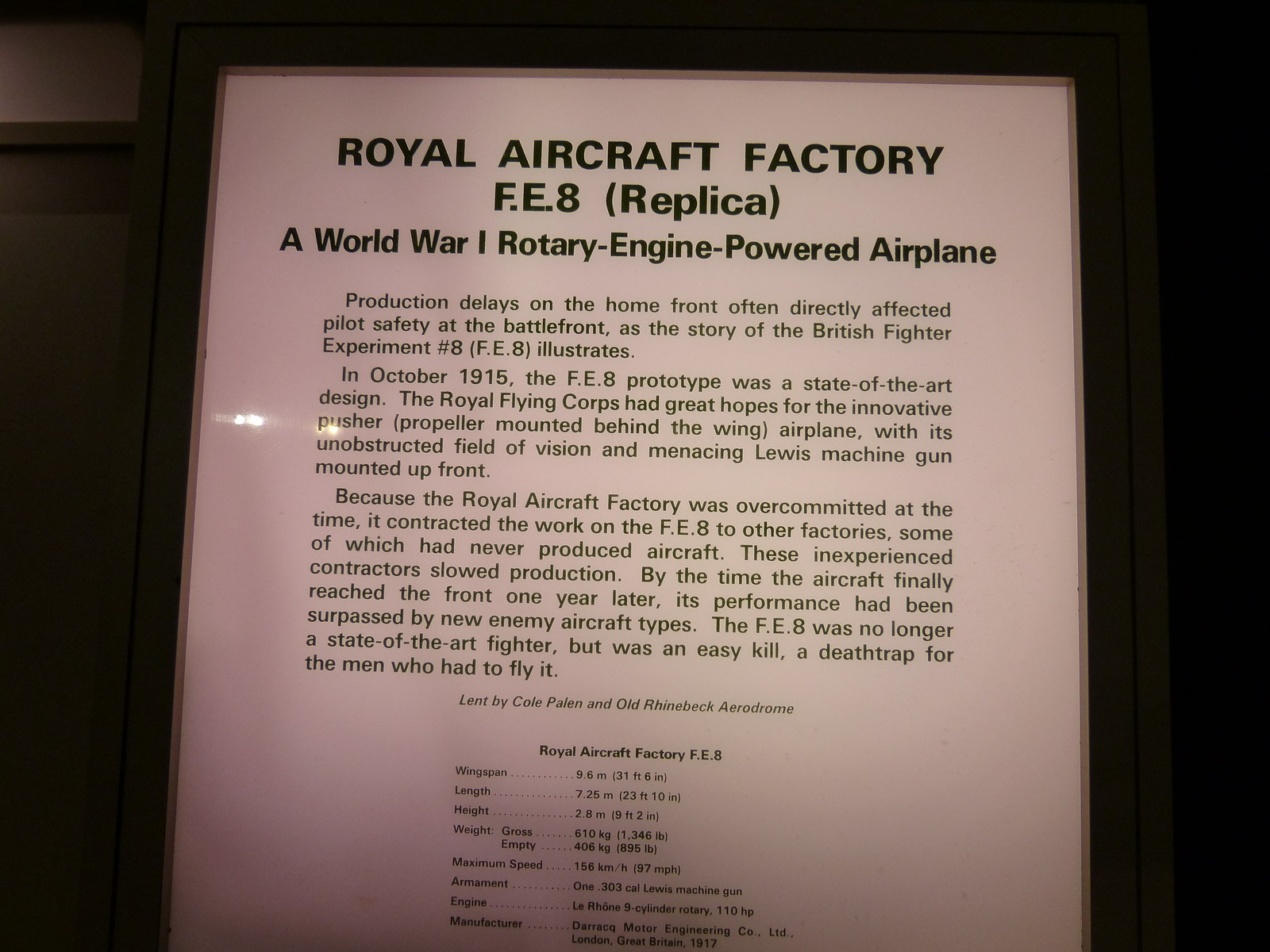The image displays a white laminated document set against a dark black background that obscures the surroundings, possibly making it appear as though it’s against a wall or in a frame. This document prominently features in bold letters at the top: "Royal Aircraft Factory FE8 (Replica)," followed by a description identifying it as a "World War I rotary engine powered airplane." The body of the text narrates the history and impact of the FE8 prototype, stating: "Production delays on the home front often directly affected pilot safety at the battlefront, as the story of the British fighter experiment number 8 (FE8) illustrates. In October 1915, the FE8 prototype was a state-of-the-art design. The Royal Flying Corps had great hopes for the innovative pusher propeller mounted behind the wing airplane, with its unobstructed field of vision and menacing Lewis machine gun mounted up front. However, because the Royal Aircraft Factory was overcommitted, it contracted work to other factories inexperienced in aircraft production, leading to slowed production. By the time it reached the front a year later, newer enemy aircraft had rendered it obsolete, turning it from a cutting-edge fighter into a death trap for its pilots." Additional details and measurements about the aircraft are found in smaller print at the bottom of the document.